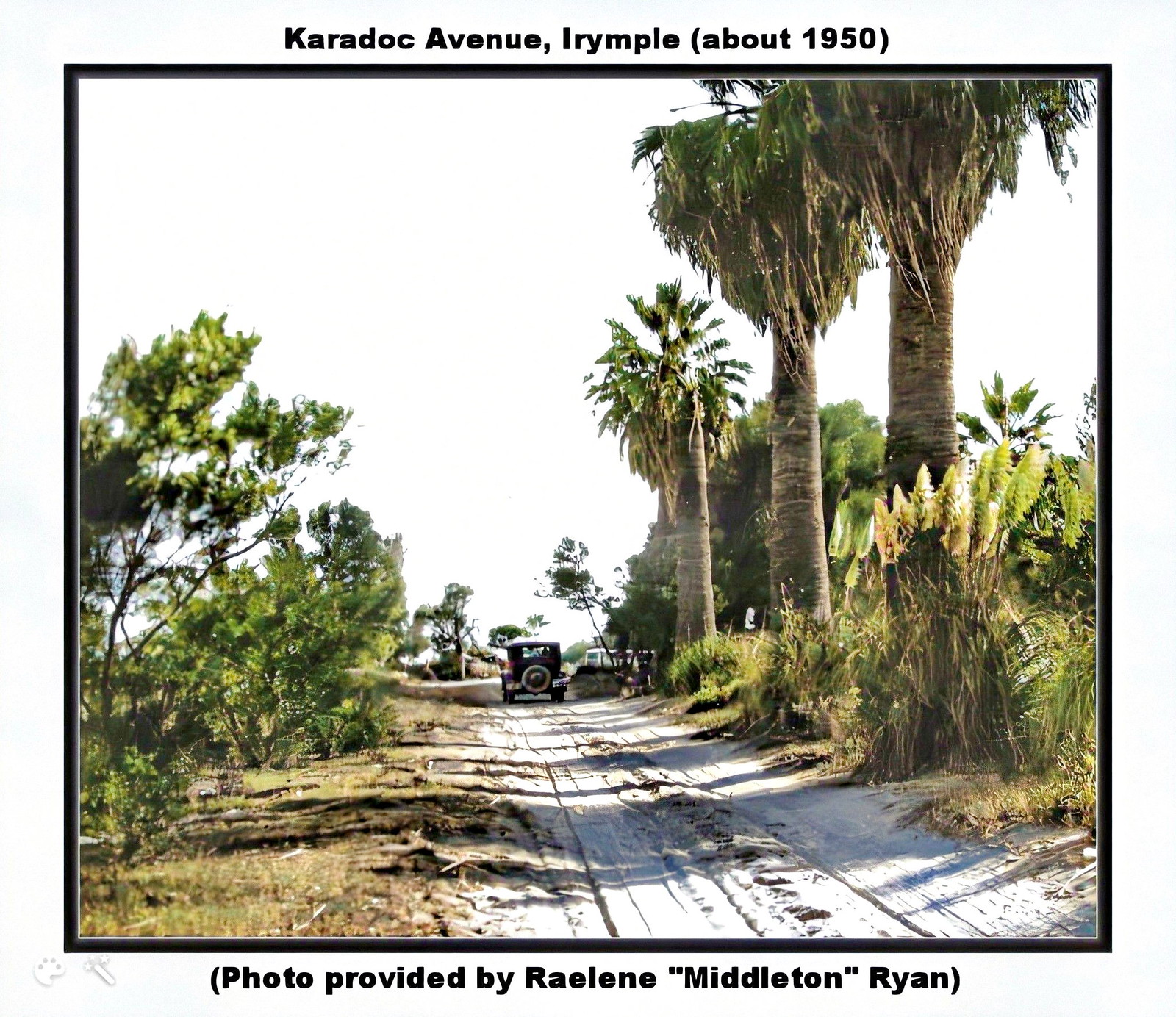This photograph, approximately 5x5 inches with a black border and nearly square in shape, depicts an old-fashioned car, reminiscent of a Model T Ford, driving down a sand-covered, primitive road. The road appears to be part of a beach, suggested by the tall, thick palm trees with visible trunks and lush palms, lining the right side. Some flowers grow around the bases of these trees. On the left side of the road, the landscape is swampy with muddy, brown grass. The road extends into the background, where a structure is faintly visible on the right. In the sky above, the overcast conditions create a bright, white expanse devoid of clouds or sunshine. Text above the photograph reads "Karadoc Avenue, Irymple, about 1950," while below, it credits "Photo provided by Raylene 'Middleton' Ryan."